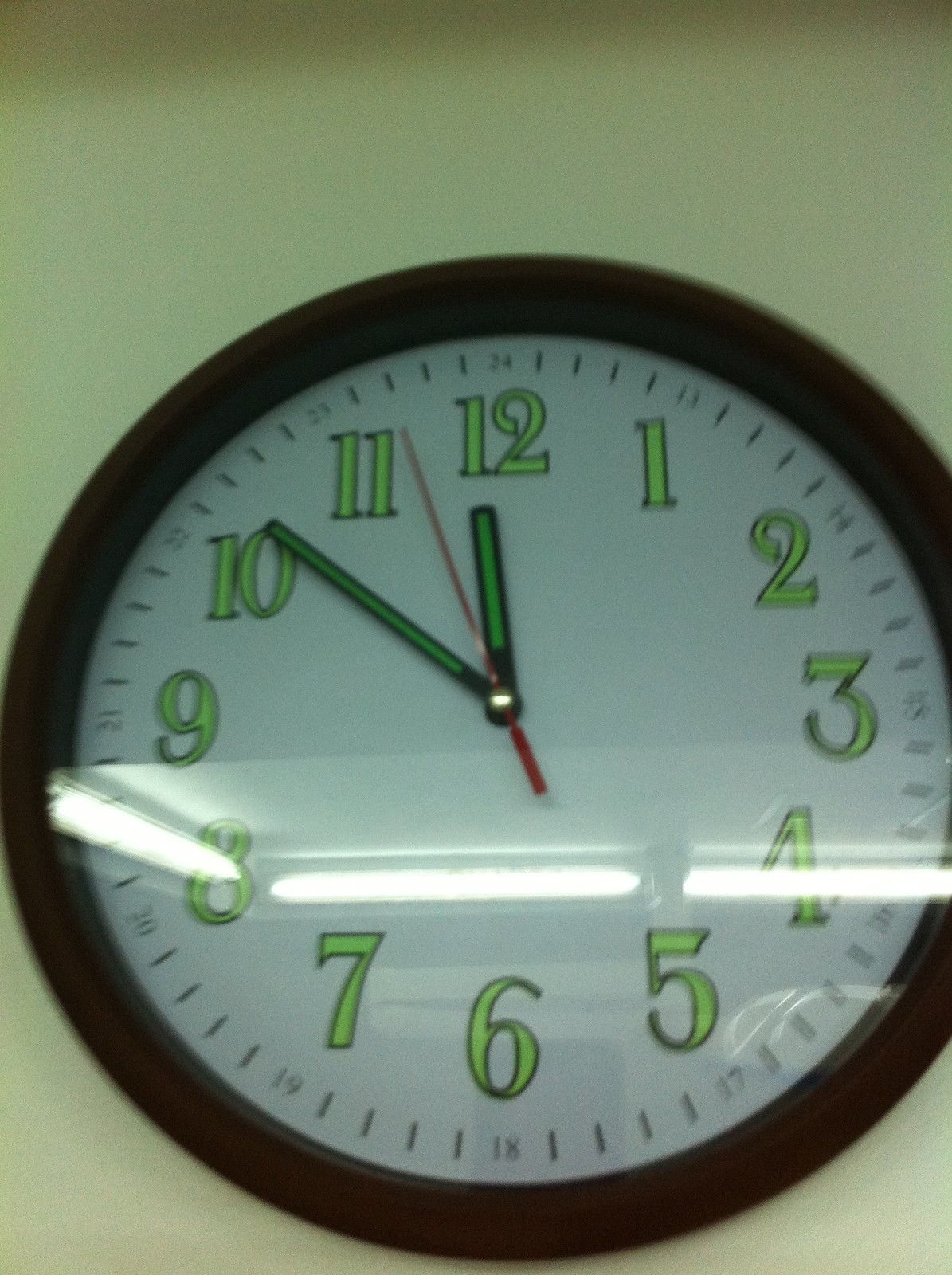The photograph captures an indoor setting, possibly an office or a school, with a clock mounted on a yellowish, off-yellow wall. The wall clock has a dark walnut brown or black wooden frame and is protected by a glass cover that reflects light from recessed lamps overhead. The clock's face is white, featuring bright neon green numbers that might glow in the dark. The minute and hour hands are black with neon green strips, presumed to be luminescent, while the red second hand adds a contrasting detail, all anchored by a small silver or gold brass screw. The time on the clock shows approximately 11:51 or 11:52. The clock's digits range from 1 to 12 in a clockwise direction, and minute markers are denoted by small black dashes.